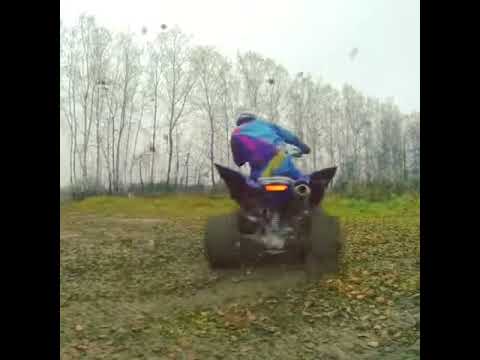The image is a wide rectangular photograph with thin black rectangles cropping the left and right sides, making the main image square-shaped. It captures the back view of a person riding a quad bike away from the camera over a green, grassy area strewn with green and brown leaves. The quad bike is blue with a red taillight, chunky squared rear wheels, an exhaust, and wing-shaped mudguards. The rider is dressed in a long-sleeve, multicolored shirt featuring stripes of turquoise, pink, yellow, and purple. They are leaning slightly to the left with their right arm visible on the handlebar, while the other arm is obscured by their body. The ground underneath the bike appears muddy with leaves scattered around, some of which are thrown into the air by the movement of the bike. In the middle of the image, at the horizon line, there is a row of very tall trees, devoid of leaves, standing against a mostly white sky that fades to a light blue in the right corner.